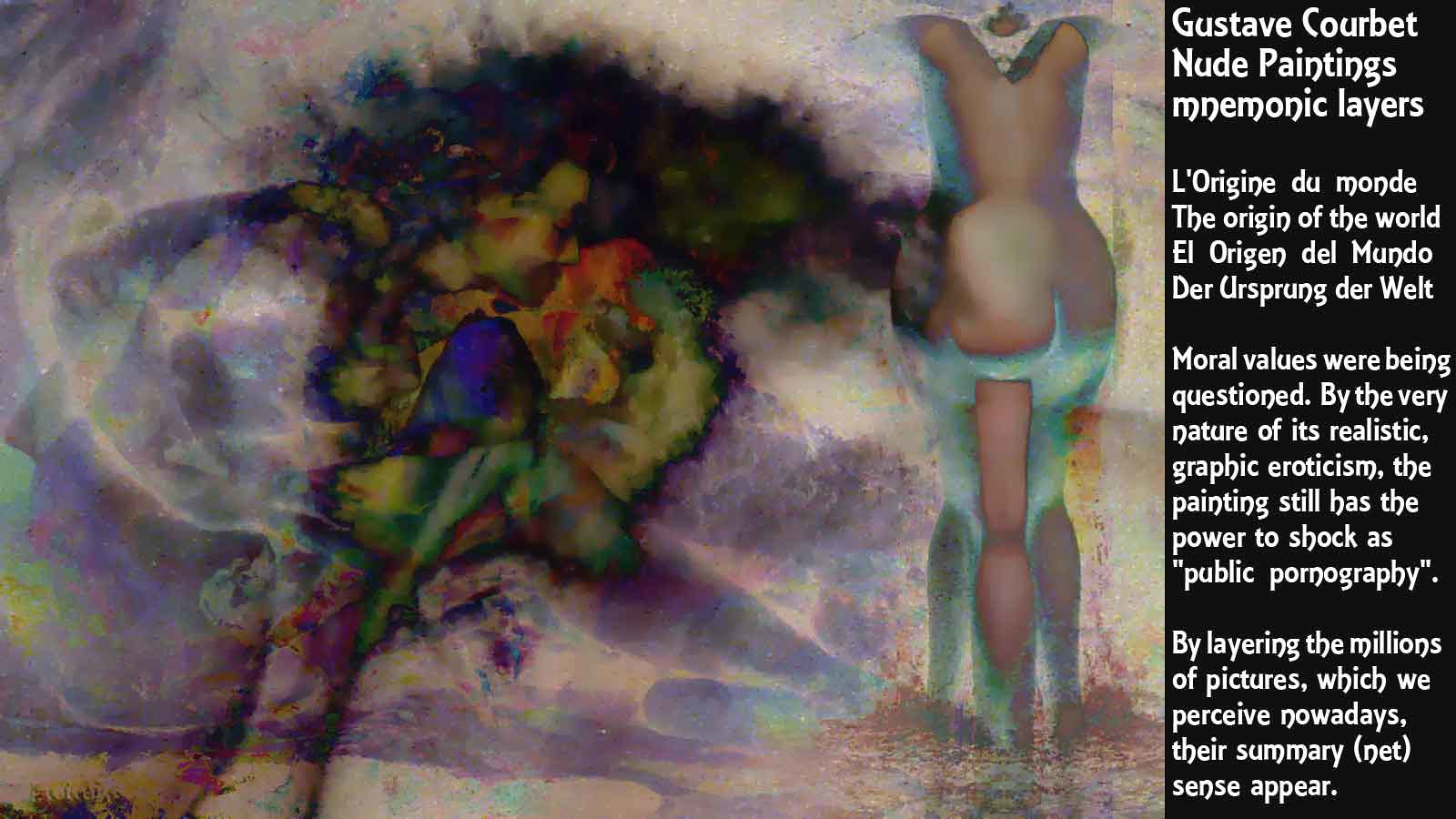The image is a detailed composite artwork titled "Nude Paintings, Mnemonic Layers" by Gustave Courbet. This piece integrates various paintings layered upon each other to evoke a psychedelic, fractal-like effect. Dominated by blobs of vibrant colors such as greens, blues, dark reds, and whites, it appears almost as a negative image due to the contrasting color tones. Notable elements within the complex layering include fragmented depictions of nude female forms, such as a woman's face and an incomplete figure of a nude woman, both rendered in muted greens and purples. The painting's right side features Courbet's name and the title, along with text in multiple languages. One such paragraph states, "By layering the millions of pictures which we perceive nowadays, their summary net sense appeal," reflecting on the provocative nature of Courbet's work and its commentary on public perception and moral values.